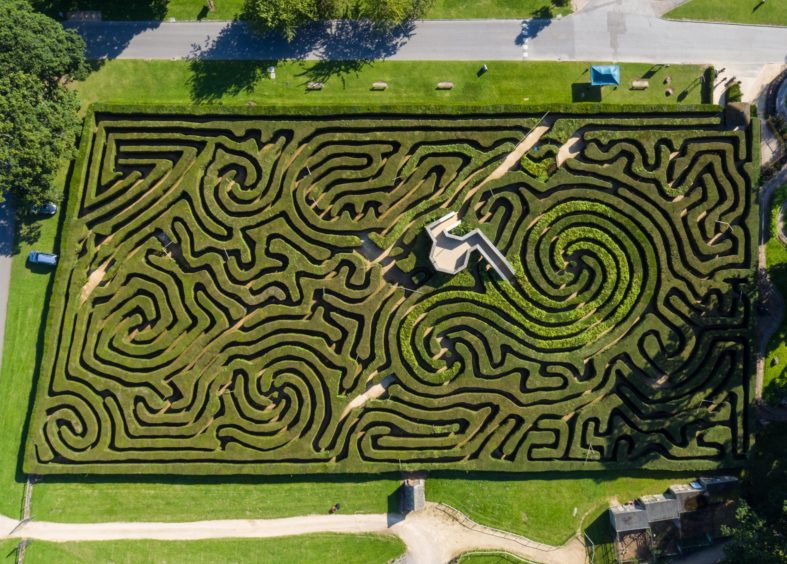This detailed aerial view showcases a large, intricate hedge maze sprawled across a green lawn, seemingly located within a park. The maze's dense, green hedges form a complex network of pathways, some of which appear to be lined with sand or dirt. In the center of the maze stands a prominent gray structure, likely an observation deck or lookout post, enabling visitors to oversee the maze and perhaps assist in finding lost companions. Surrounding the maze, the scene includes various elements: grassy borders, multiple sidewalks, and scattered structures such as buildings or sheds, possibly a tent and some rocks. Along the top of the image, a roadway can be seen with vehicles parked on the left side, while the bottom edge reveals a few houses and another road. Despite the elaborate design, no people are visible within the maze at this time, emphasizing its vast and tranquil layout.